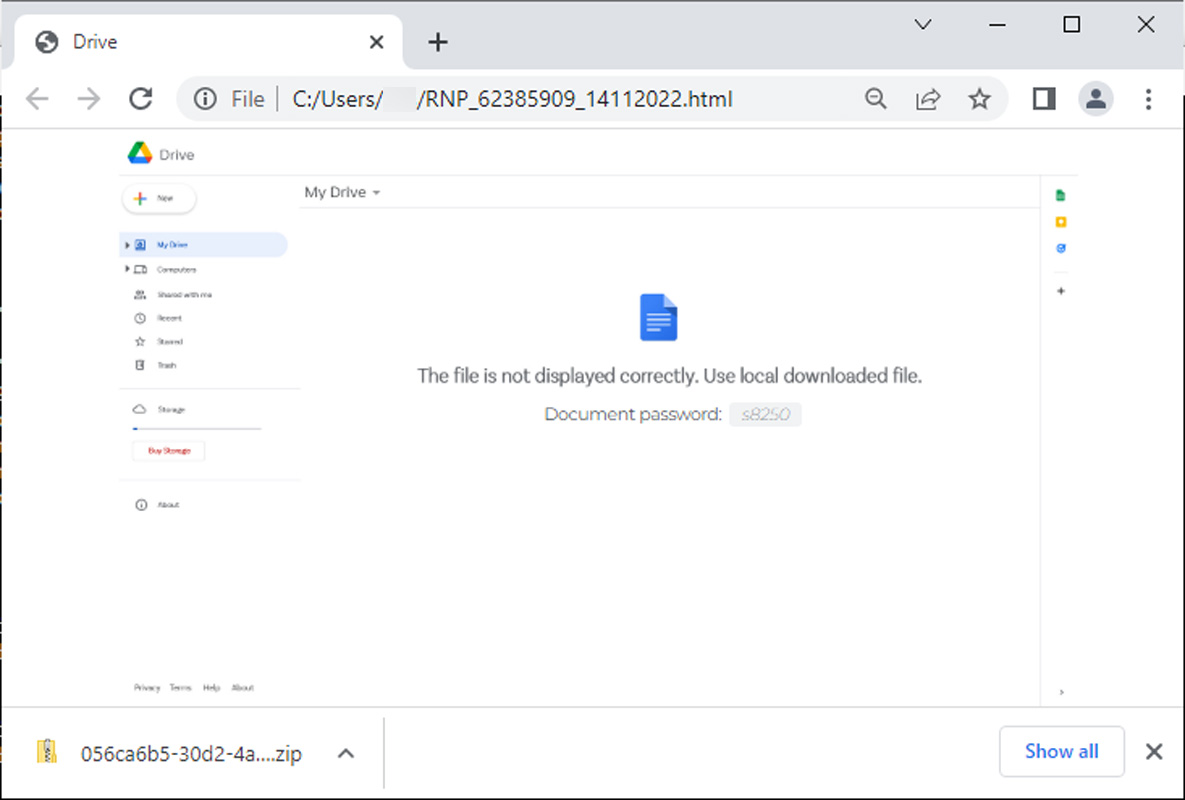This image captures a screenshot of a Google Drive webpage. At the top of the browser, the word "Drive" is displayed next to a black and white circle icon. The website's header features a gray background with a navigation path that reads "file / C: / users / [blank] / RNP," followed by an extensive string of numbers. 

Directly beneath this path is the Google Drive logo, a colorful triangle, with the word "Drive" beside it. Adjacent to this, there's a "New" button accompanied by a Google-colored plus sign. 

The main content area displays the "My Drive" section, where a blue icon depicting a piece of paper with its right corner folded down is visible. The icon has white horizontal lines, resembling a document. A message on the document states, "The file is not displayed correctly. Use local downloaded file. Document password: 8250."

On the left-hand side of the webpage, a navigation menu lists various categories. The highlighted category, shaded in blue, appears to be labeled "My System" or something similar, with a blue icon next to it. The remaining categories are listed in black text. One section stands out in red lettering. At the bottom of the menu, there's a blue "Show All" button.